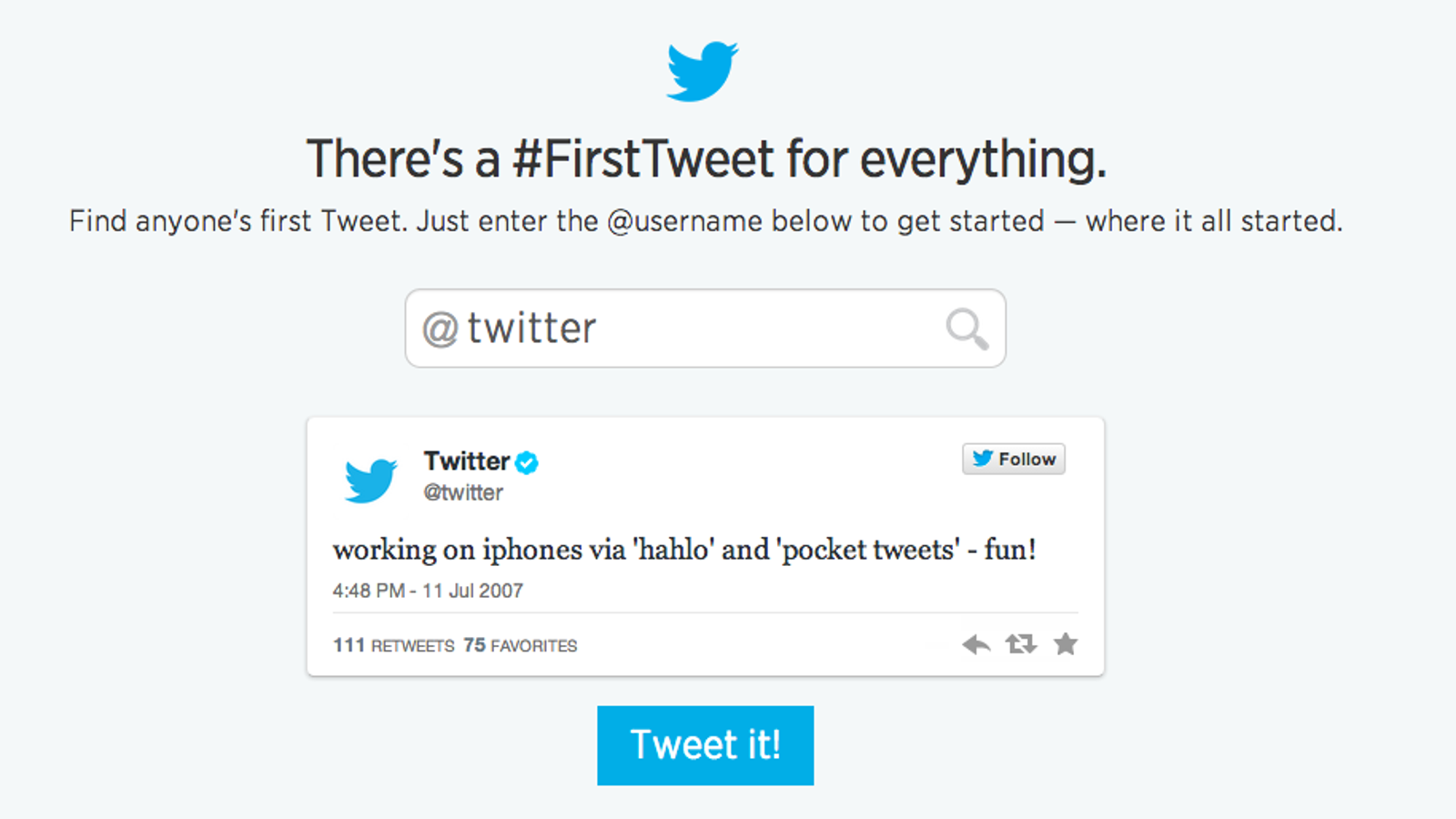The image depicts an entry screen for Twitter. At the pinnacle of the screen, prominently displayed is the iconic Twitter logo, featuring the little blue bird. Underneath the logo, a caption in black font declares, "There's a first tweet for everything," with the hashtagged phrase "#FirstTweet" seamlessly embedded within. Further down, instructional text invites users to "Find anyone's first tweet. Just enter the username below to get started."

Positioned below these instructions is a text box designated for entering a Twitter username. Within this box, the username "Twitter" has already been inputted. Subsequently displayed is the inaugural tweet by Twitter itself, which succinctly states, "working on iPhones," and is timestamped July 11, 2007. Directly beneath this display, a light blue button is prominently positioned, featuring the prompt "Tweet it" in crisp white text.